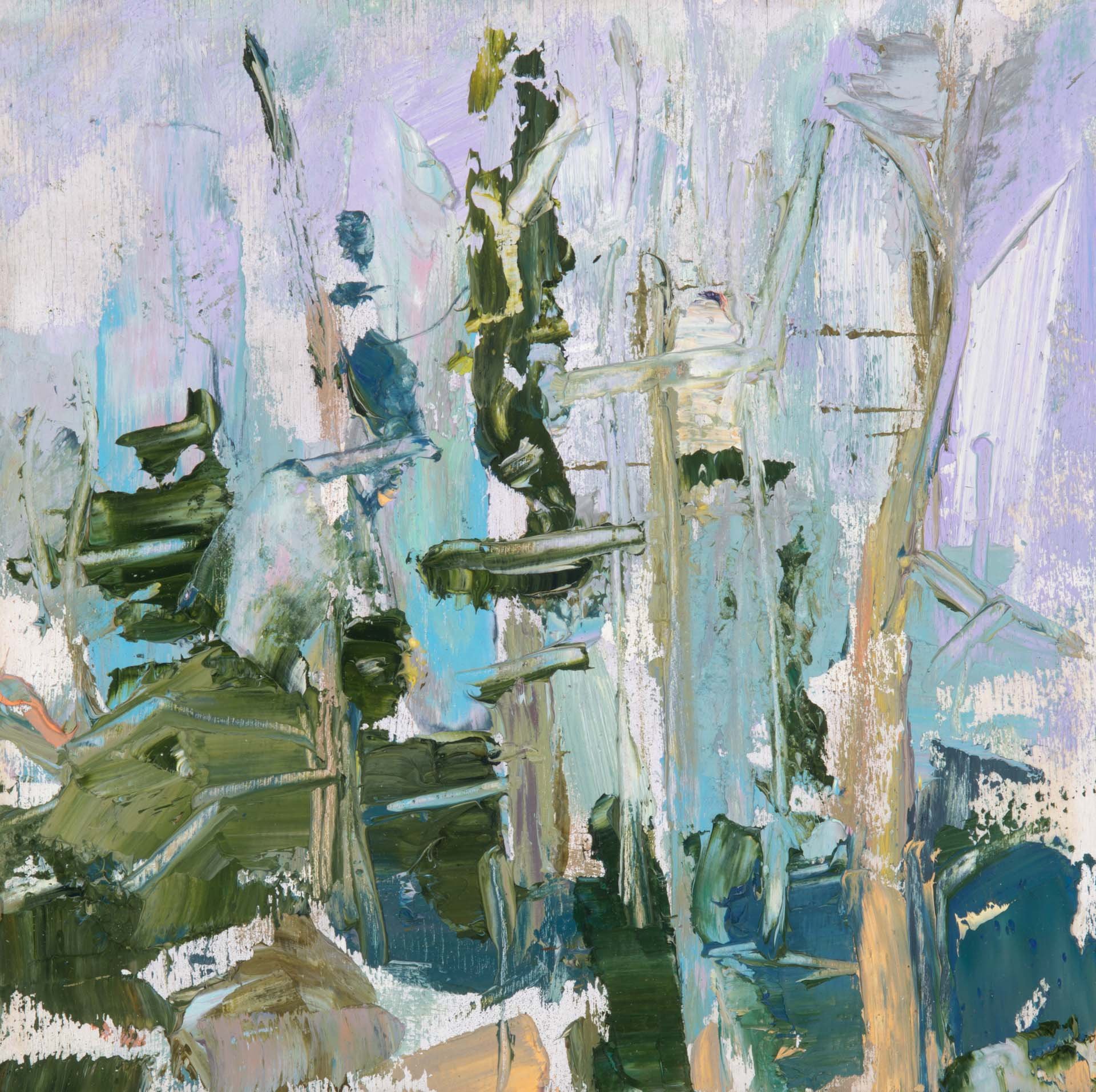This image is a painting, likely an abstract or impressionist piece, dominated by flowing brushstrokes and a blend of vibrant colors. Central to the artwork is a statue-like figure with a predominantly green base, transitioning into yellow around the body, and capped with green paint that suggests hair. Adjacent to this statue is a tan, leafless tree that adds to the abstract landscape's enigmatic quality. The painting features a rich palette, with dominant shades of lavender in the top right corner, melding into greenish-blue hues toward the bottom right, and further transitioning into lighter shades of white and lavender. The bottom left corner of the canvas is rich with darker greens and browns, hinting at a hilly terrain. This evocative use of color and form likely interprets a surreal landscape teeming with trees and natural elements, though its abstract nature leaves room for varied interpretation.